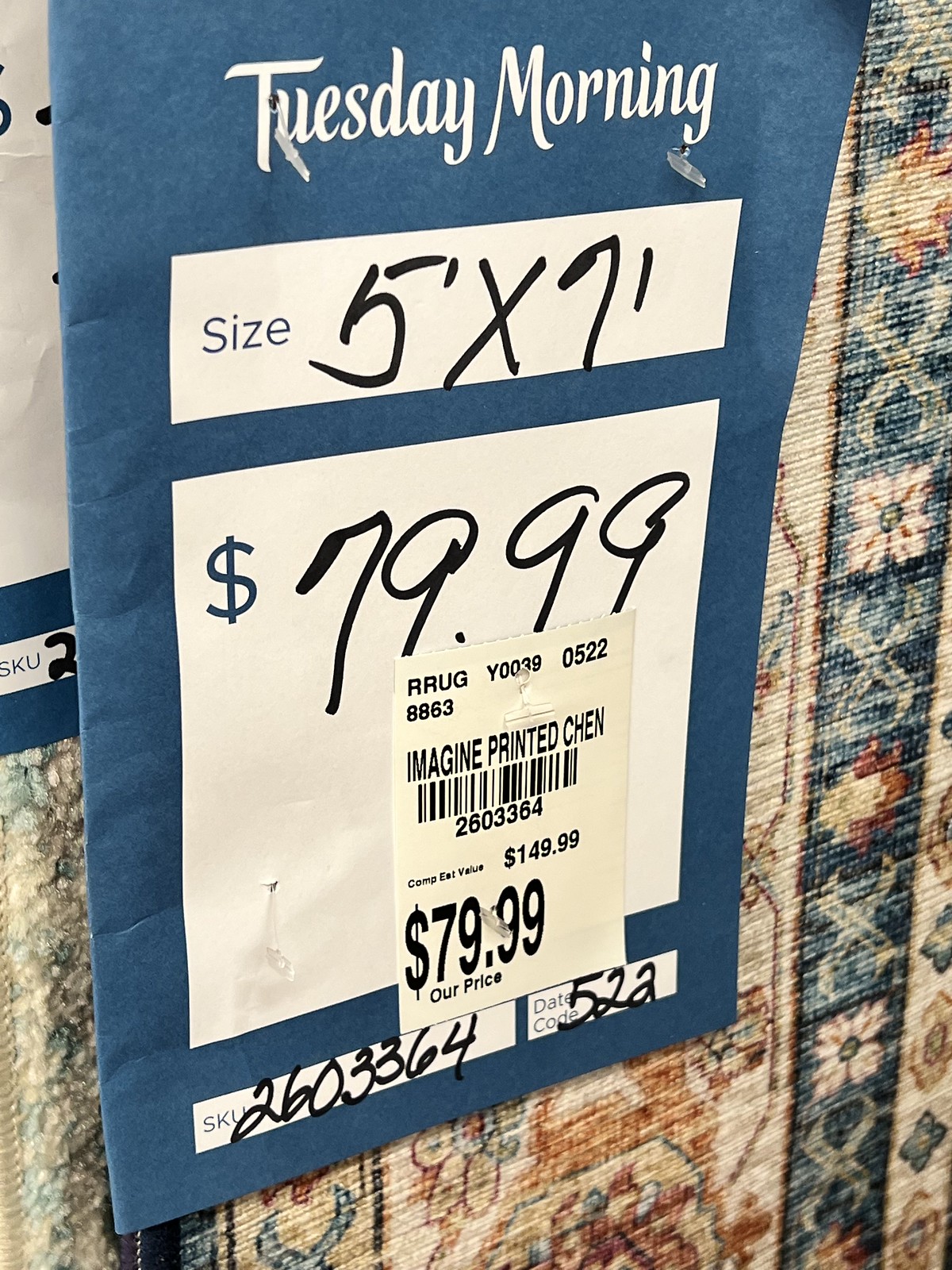The image depicts a vertically-oriented photograph of a rug flipped upside down, displayed in a store. The rug's backside, revealing its less attractive weave, is predominantly beige with a vertical teal stripe featuring floral patterns and additional brown designs throughout. A blue sign, attached to this tapestry-like rug, faces approximately four o'clock. The royal blue sign states "Tuesday Morning" in white text and indicates the rug's dimensions as "5x7 feet." The rug is priced at $79.99, with a SKU number 2603364 and a UPC code visible at the bottom. The printed sign appears to be stuck to the rug's surface, adding a layer of retail detailing to the overall presentation.